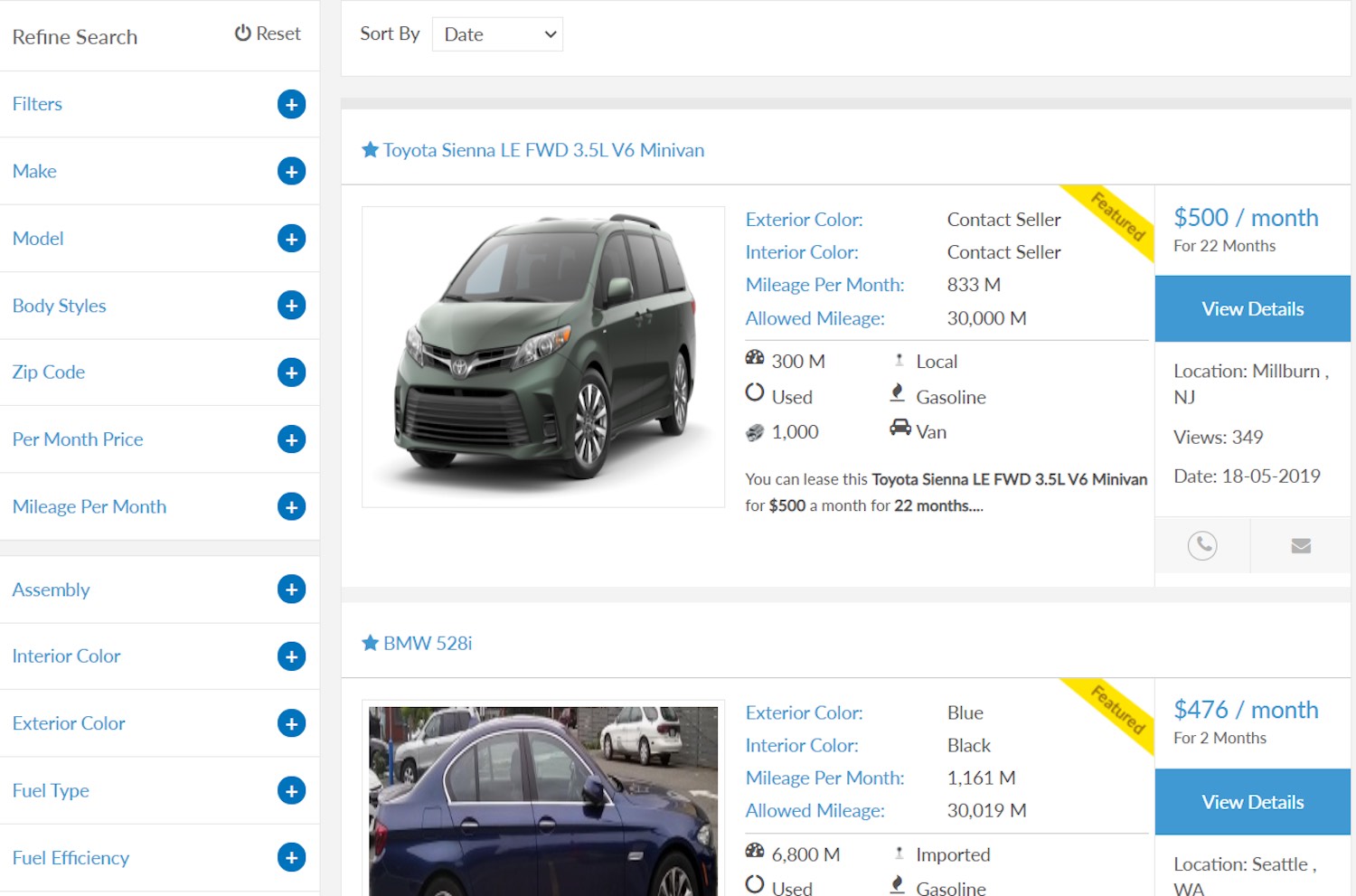On the left side of the image, there is a large menu titled "Refined Search" in black text at the top. Towards the right of this title, there is a power button symbol—a circle with a break at the top center and a line through it. To the right of this symbol, in dark gray text, it reads "Reset."

Each menu option is separated by a gray dividing line. To the right of each option, there is a dark blue circle with a white plus sign in its center. The menu options are listed in blue text in a basic sans-serif font. They are as follows: Filters, Make, Model, Body Styles, Zip Code, Per Month Price, and Mileage Per Month. Following a small break in the menu, additional options are listed: Assembly, Interior Color, Exterior Color, Fuel Type, and Fuel Efficiency. The menu is cut off at this point, so additional options, if any, are not visible.

To the right side of the image, there is a white header with "Sort By" written in black on the left. Next to this, there is a dropdown menu with a white background and "Date" written in black, accompanied by a black arrowhead indicating a dropdown function.

Below the header, there is a rectangular area with a white background. In the upper left corner of this rectangle, there is a filled blue star and the text "Toyota Sienna LE FWD 3.5L V6 Minivan" written in blue. Beneath this text, an image of the minivan in forest green color is displayed.